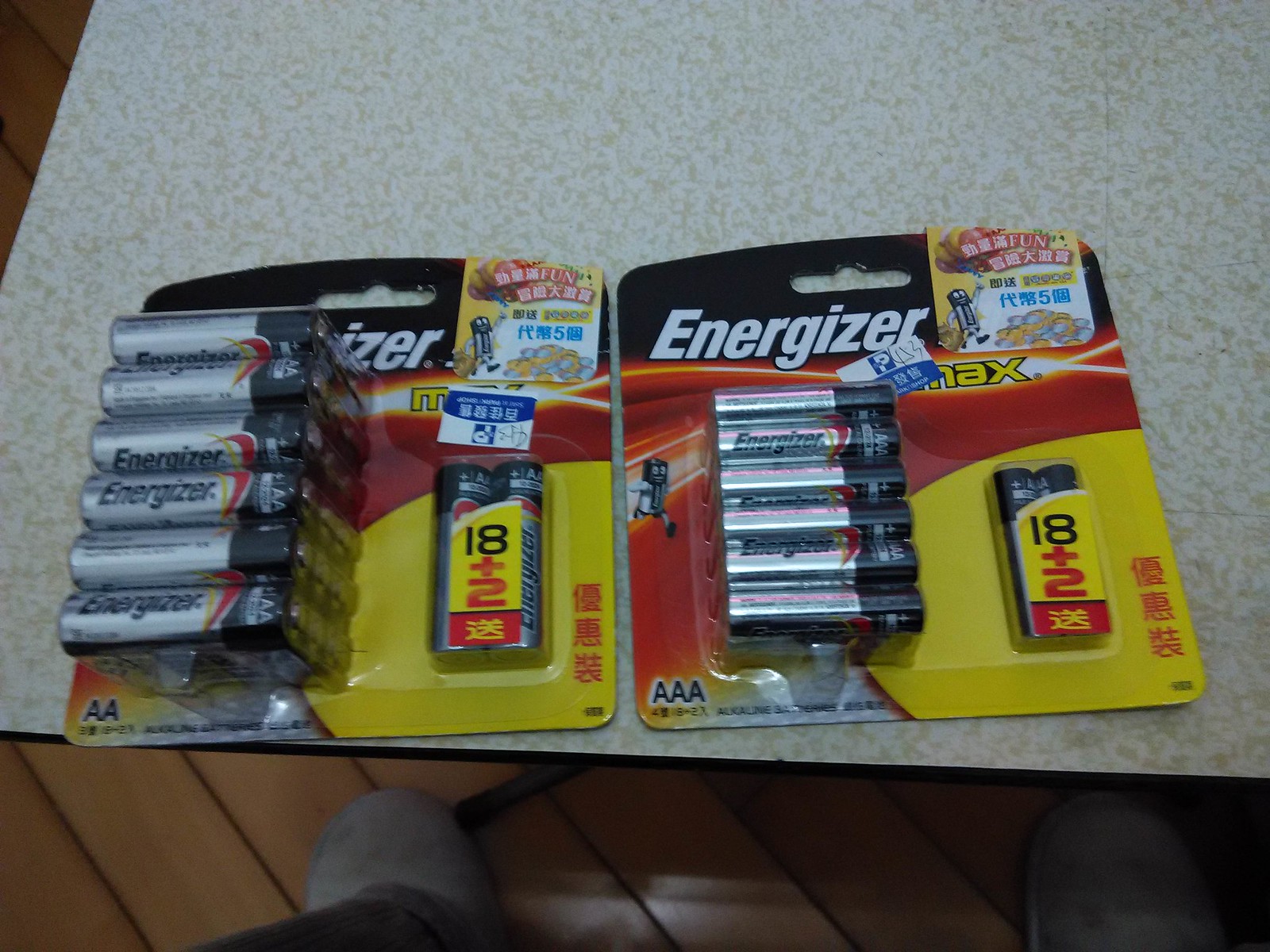A detailed photo captures two unopened promotional packs of Energizer Max batteries displayed on a cream and gold modeled laminate table. A pair of gray shoes and dark pants, belonging to the person taking the picture, are also visible against the wooden floor in the foreground. The pack on the left contains AA batteries, while the pack on the right holds AAA batteries. Each pack includes a total of 20 batteries, comprising 18 regular plus 2 free ones, clearly marked with "18 + 2" promotional signage. The battery packaging features a design of yellow, red, and black with white lettering, and includes text in an Asian language, possibly Japanese or Chinese. The image is likely taken for resale purposes, such as on Facebook Marketplace or Craigslist, and the batteries are in their original blister packaging typically found hanging in stores.